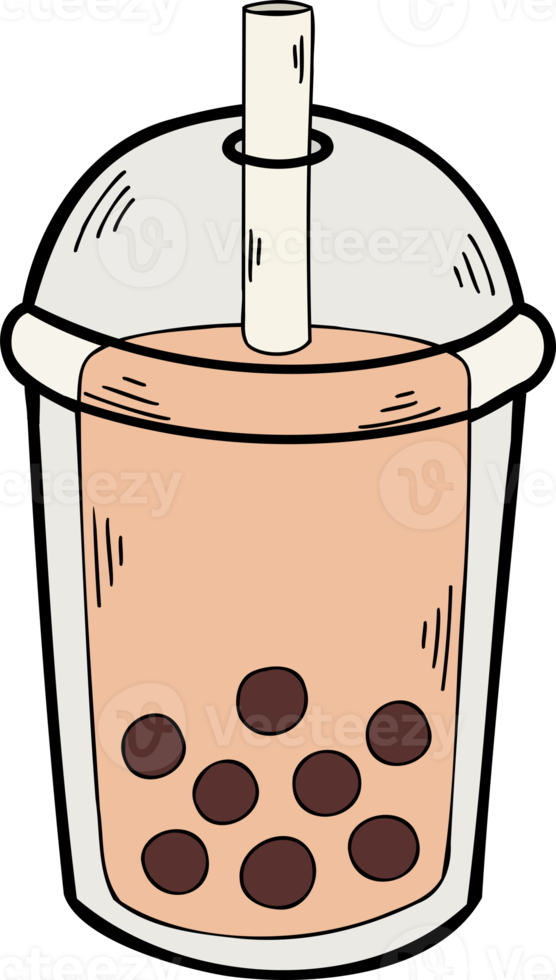This is a digitally created image on a white background, featuring a translucent cup with a bubble lid and a straw inserted at the top. The cup appears to be hard plastic and has a light blue tint with a liquid inside. The liquid is pinkish, and within it, there are several ice cubes or pieces of fruit, which are apricot beige in color and have dark brown circular spots or holes. The cup is detailed with multiple black lines outlining it horizontally and vertically, adding a stylized touch. Additionally, the image has a watermark that says "Vecteezy" in gray or white letters.